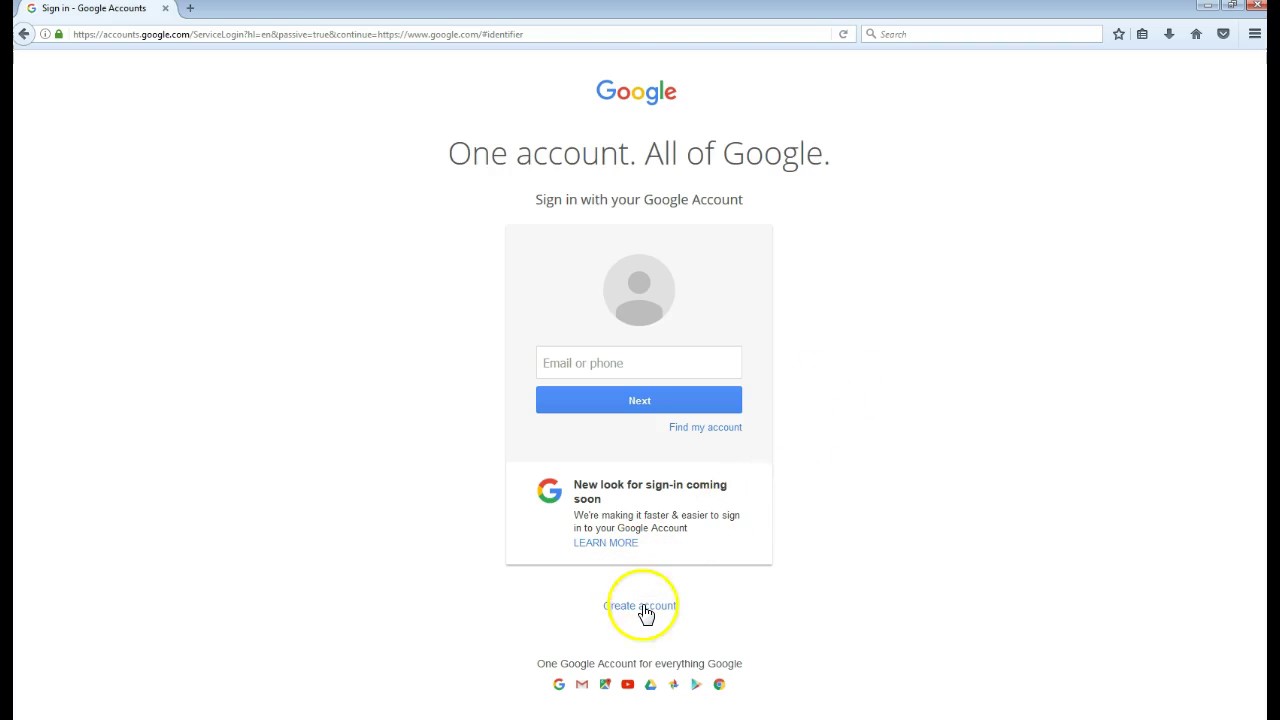A computer screen displays a Google Accounts sign-in page open on a web browser. The browser shows only one tab, which is securely connected via HTTPS, indicating with a green padlock icon in the URL bar: https://accounts.google.com followed by a string of characters. At the top of the webpage, the header reads "Sign in – Google Accounts."

In the center of the page, the colorful Google logo stands prominently, just above bold text that states, "One account. All of Google." This section invites the user to sign in with their Google account.

Below this, there is a white input field with a silhouette of a person icon inside a circle, labeled "Email or phone." Adjacent to this input field is a blue "Next" button. Below this option is a smaller link labeled "Find my account."

Further down, a notice represented by a capital "G" informs users of a "New look for sign in coming soon."

At the very bottom of the screen, the text "Create account" is highlighted with a yellow circle, and an animated white-gloved hand points towards it, emphasizing the option for new users to create an account.